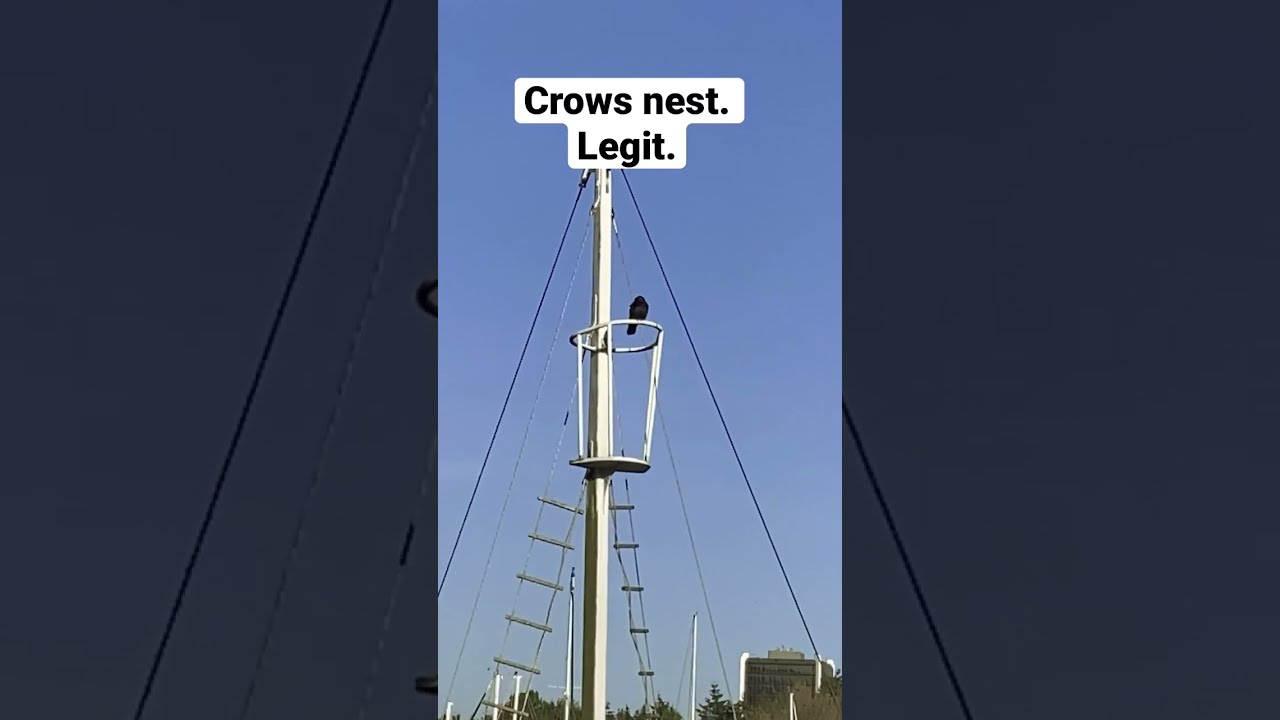This vertical, portrait-style photograph captures a tall, white mast extending upwards from the bottom of the frame, set against a clear blue sky. This mast is adorned with rope ladders on either side and features various cables running down likely for sail adjustments. Near the top of the mast is a small, one-person platform resembling a crow's nest, encircled by three to four vertical metal bars. Perched on this railing is a black crow. The background shows faint treetops and distant masts from other boats, enhancing the nautical atmosphere. Overlaid on the photo is a white bubble with black sans serif text that reads "crow's nest. legit."